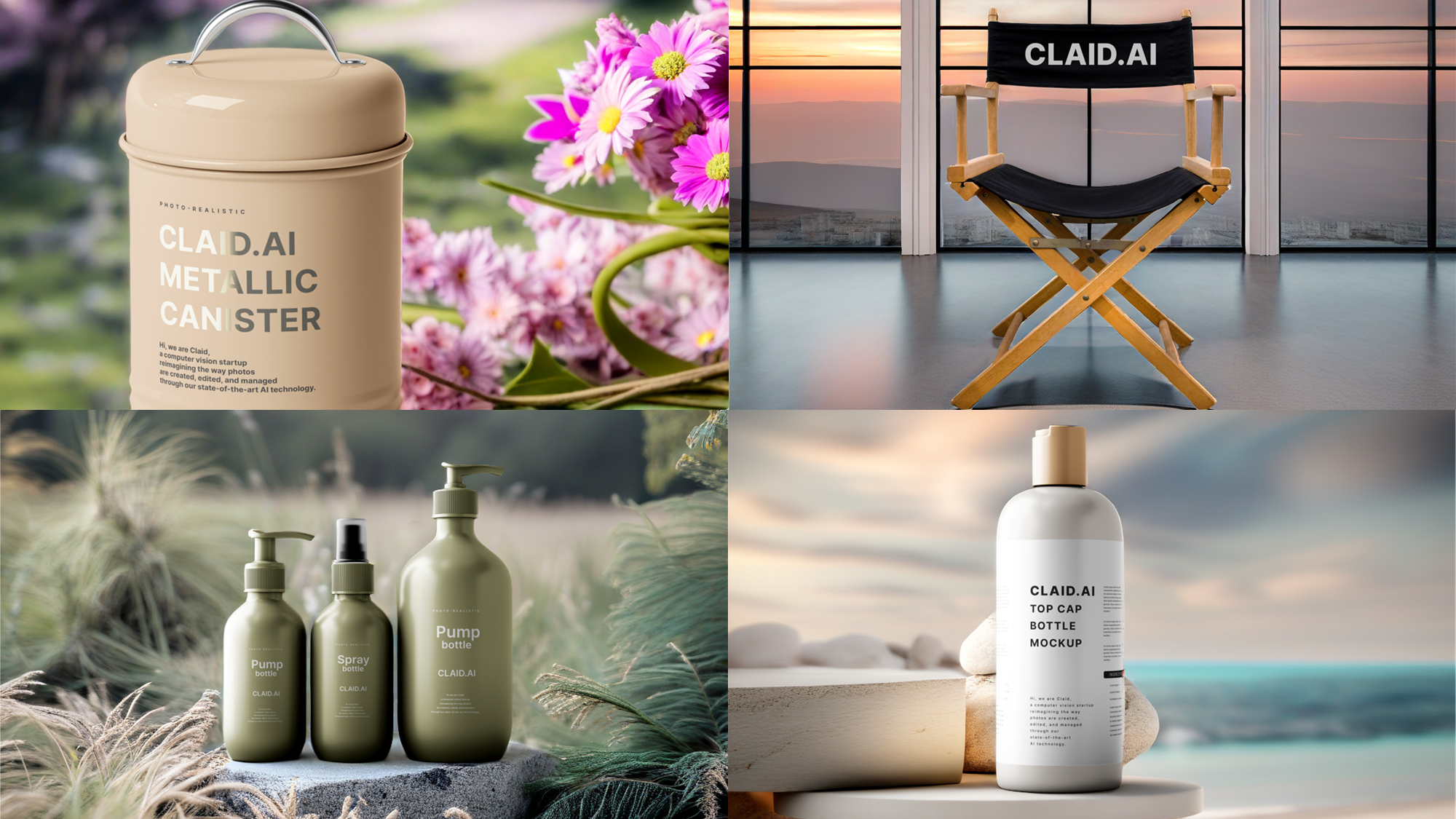The image, featuring a horizontal layout composed of four equally-sized, professionally-staged photographs, showcases various products from the company clad.ai. In the upper left-hand corner, a beige metallic canister labeled "clad.ai" is set against an outdoor backdrop with purple and pink flowers, and hints of a steer's horns depicted on the can. Moving to the upper right-hand corner, a black wooden director's chair with a light wood frame prominently displays "clad.ai" across its fabric backrest. This chair is positioned in front of a large window that reveals a hazy mountain landscape bathed in orange sunlight. The bottom left-hand corner highlights three greenish, furry-textured pump containers placed on a gray stone amidst a grassy field, reflecting an earthy, natural theme. Lastly, the bottom right-hand corner shows a sleek white squeeze bottle with a gold cap, also marked "clad.ai," set against a serene seascape background. Together, these images collectively represent the diverse range of clad.ai's product concepts with an emphasis on natural elements and sleek design.